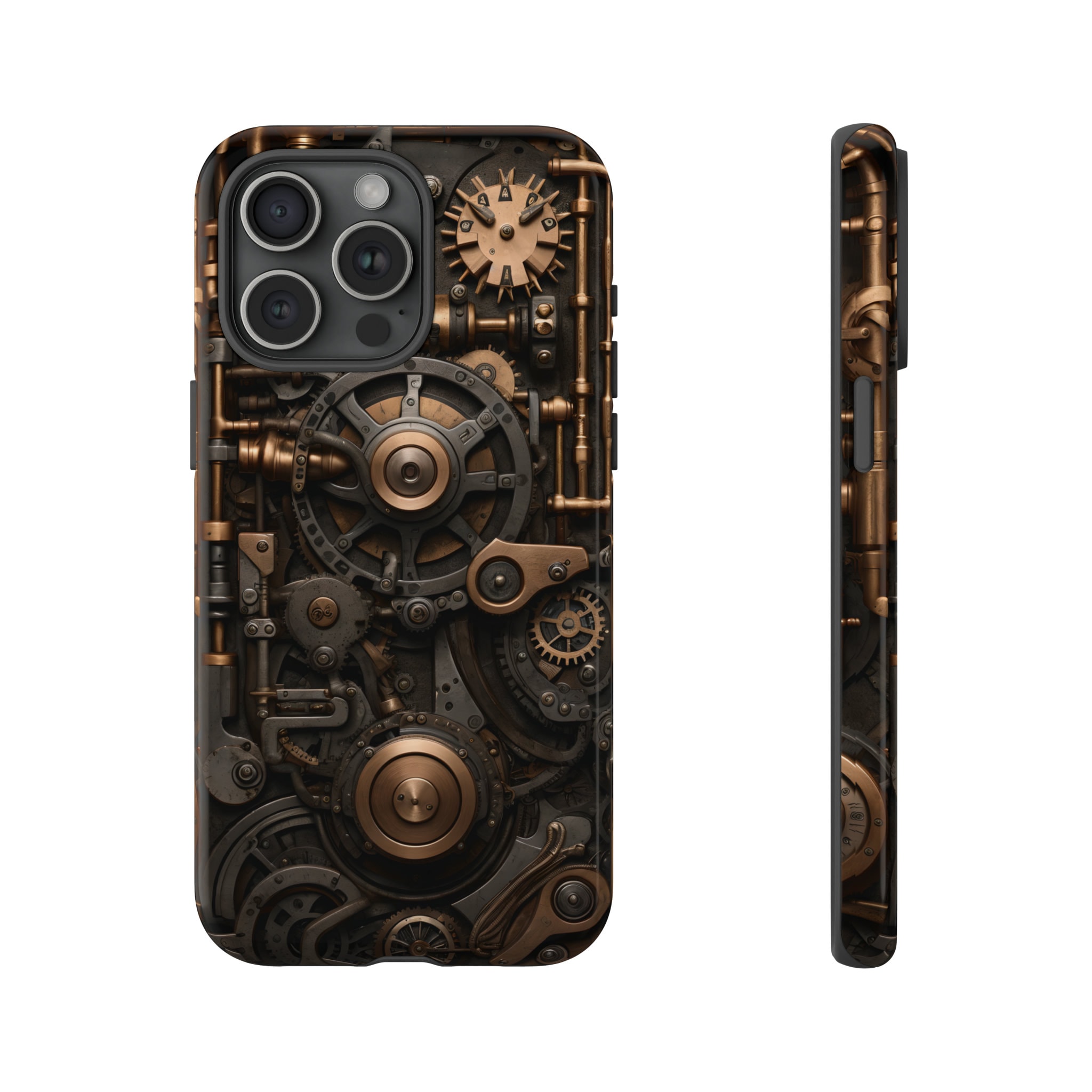This image showcases a product photograph of a protective case for a mobile phone, likely an iPhone, adorned with an intricate steampunk design. The composition features two side-by-side views against a blank white background: a full back view and a slender side profile. The phone case itself, made from solid plastic, is characterized by a detailed pattern of interlocking gears, mechanical piping, and levers, rendered in dark brown, bronze, and black hues to create a highly metallic and almost three-dimensional effect. Prominent elements include two large gears at the lower portion and one spiky gear in the upper right corner, with numerous connecting pipes. The back view of the case highlights a square cutout in the upper left for the camera, housing three lenses arranged in a triangular shape and two flashlights. The intricate gear design seamlessly extends across the sides, offering a cohesive steampunk aesthetic. The overall effect is a visually striking, detailed, and cool phone cover.